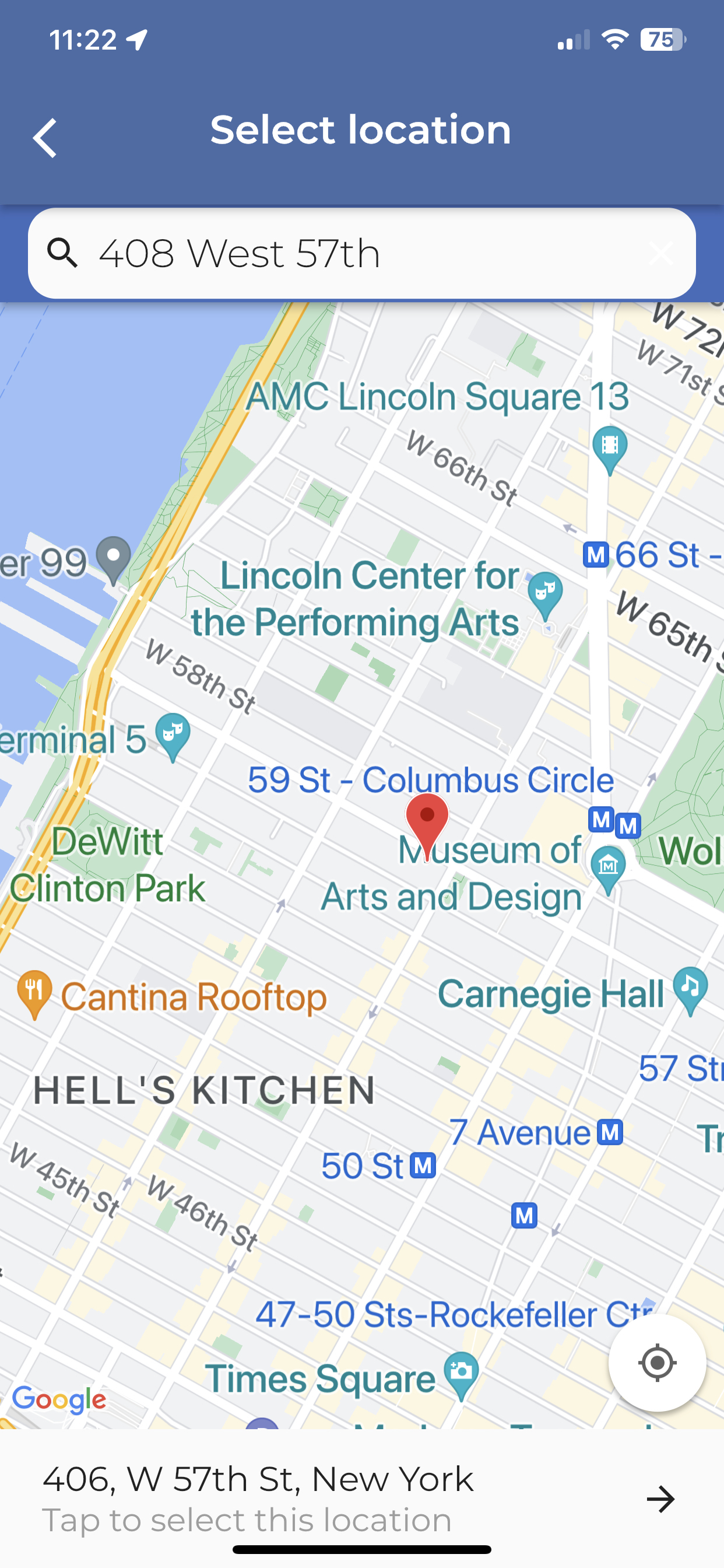In this image, a phone screenshot is displayed. At the top-left corner, the time reads 11:22, while the battery status in the top-right corner shows 75% remaining. Below these indicators, there is a navigation element with a back button to the left and the text "Select Location" at the center. Just beneath this bar, a search field contains the address "408 West 57th."

The main part of the screenshot showcases a map with a red pin marking a location near the Museum of Arts and Design. Various other points of interest are highlighted on the map, including a food symbol labeled "Cantina Rooftop" and a music symbol indicating "Carnegie Hall." The map also notes prominent areas such as Hell's Kitchen, Times Square, 47th and 50th Street, and Rockefeller Center. The upper-left portion of the map shows a body of water. At the bottom of the screen, a bar reads "406 W 57th Street, New York. Tap to select this location."